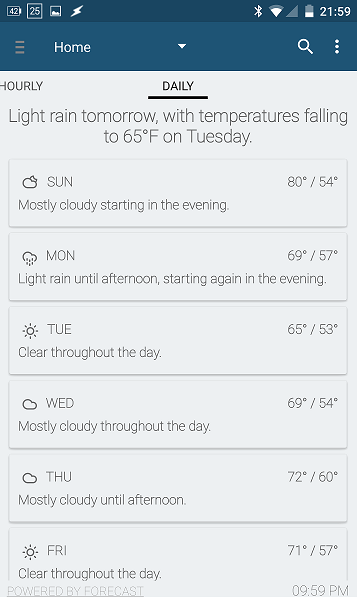A weather app interface is displayed with a blue header, featuring navigation elements including a "Home" button, a hamburger icon, a magnifying glass icon, and three vertical dots. The current time shown is 21:59. The interface includes options for "Hourly" and "Daily" forecasts, with the "Daily" tab highlighted. 

The forecast details are as follows:
- **Sunday:** Partly cloudy with some sunshine, high of 80°F and a low of 54°F.
- **Monday:** Cloudy with rain in the morning and evening, high of 69°F and a low of 57°F.
- **Tuesday:** Clear throughout the day, high of 65°F and a low of 53°F.
- **Wednesday:** Mostly cloudy throughout the day, high of 69°F and a low of 54°F.
- **Thursday:** Mostly cloudy until the afternoon, high of 72°F and a low of 60°F.
- **Friday:** Sunny throughout the day.

The forecast indicates light rain expected tomorrow, with temperatures dropping to 65°F on Tuesday.